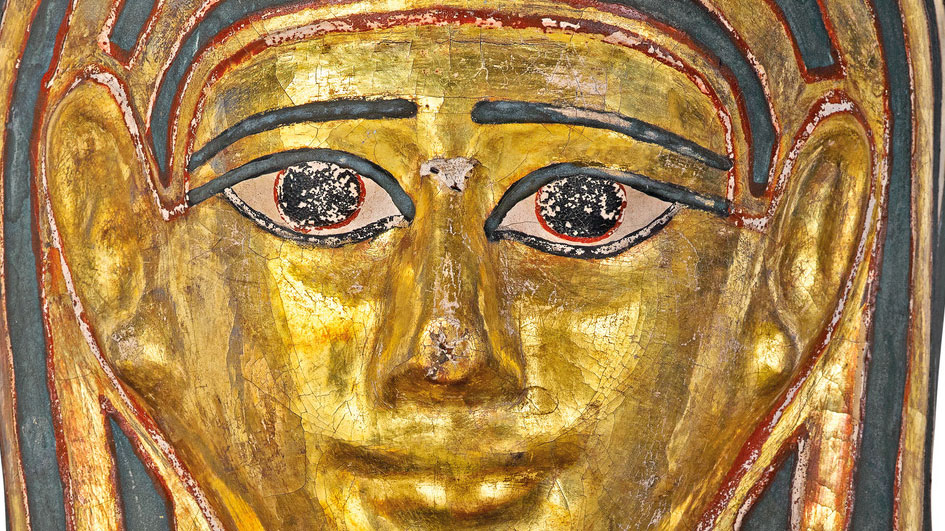This detailed photograph captures the front of an ancient Egyptian sarcophagus, showcasing a 3D face prominently gilded in gold. The face, which bears an uncanny resemblance to King Tutankhamun, features striking almond-shaped eyes highlighted with traditional Egyptian black eyeliner or kohl. The eyes are brown with white flecks and are deeply lined, accentuating the characteristic Egyptian style makeup. The eyebrows are long, fine, and dark, framing the face perfectly. The mask has large ears that jut out slightly, and the lips form a subtle smile. The headdress, adorned with blue and possibly black and red stripes, sits atop the head, adding to the grandeur of the piece. There is notable wear at the bridge of the nose, hinting at the artifact's ancient origins. The painting or photograph is horizontally rectangular and includes no visible writing, human beings, animals, or additional structures within the frame.